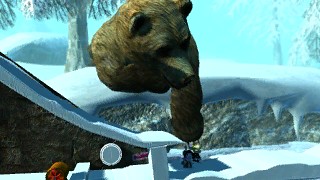In this image, we observe a computer-generated scene that might derive from a video game. The image is relatively small, necessitating a zoom for detailed observation. The background features a tranquil, snow-covered hill adorned with scattered trees. In the foreground, two diminutive characters are positioned, possibly as figures within the game. Higher on the hill, a colossal brown bear stretches towards these characters, its posture appearing non-aggressive. The bear's reach seems more inquisitive than threatening. The overall ambiance of the scene suggests a peaceful interaction amidst a wintery landscape. The image does not contain any text.